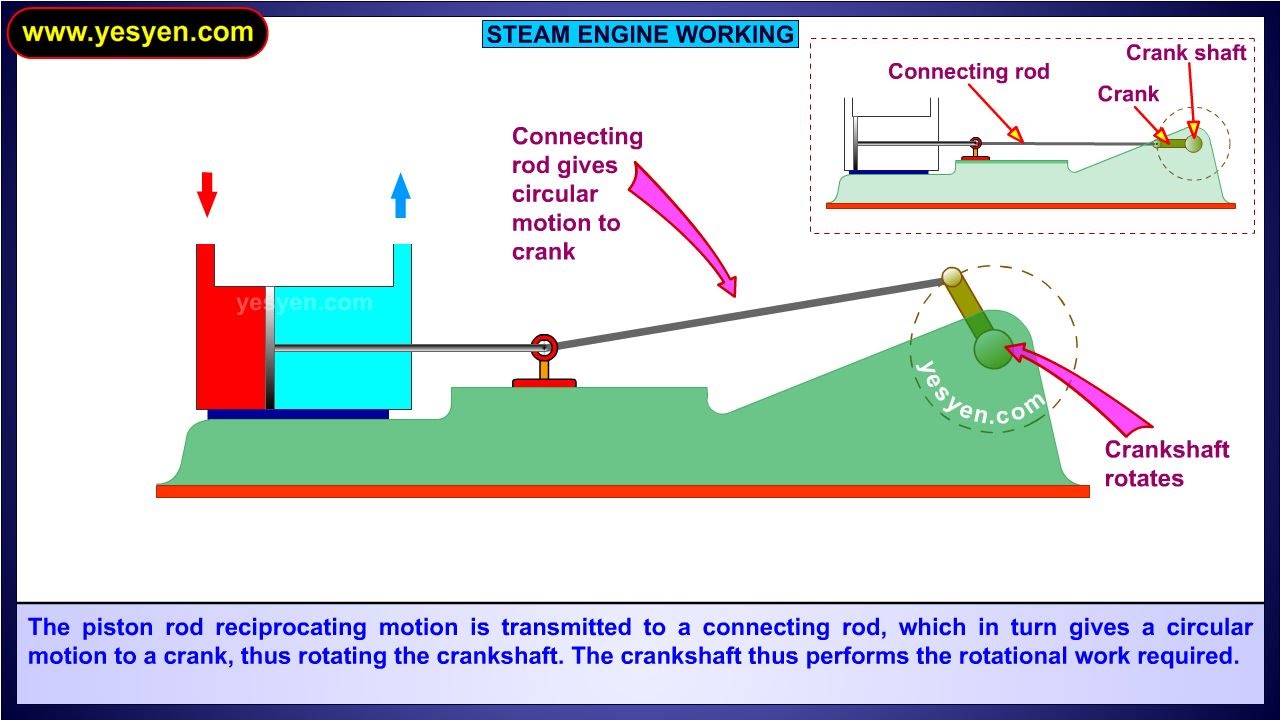This detailed diagram from yesyen.com illustrates the working mechanism of a steam engine. The main image, predominantly green with red and blue accents, visually explains how the motion is transferred within the engine. Central to the diagram is the crankshaft positioned on the right side, depicted in gray, which connects to a connecting rod. The connecting rod passes through a small opening and is essential in converting the reciprocating motion of the piston rod into circular motion, as denoted by the red arrow pointing down and the blue arrow pointing up. This circular motion subsequently rotates the crankshaft, enabling it to perform the necessary rotational work. Complementing the main diagram, a smaller image in the upper right corner provides a focused view of the crankshaft, crank, and connecting rod, further clarifying their relationship and function. The bottom of the diagram features descriptive text summarizing the process: "The piston rod reciprocating motion is transmitted to a connecting rod, which in turn gives a circular motion to a crank, thus rotating the crankshaft. The crankshaft thus performs the rotational work required."